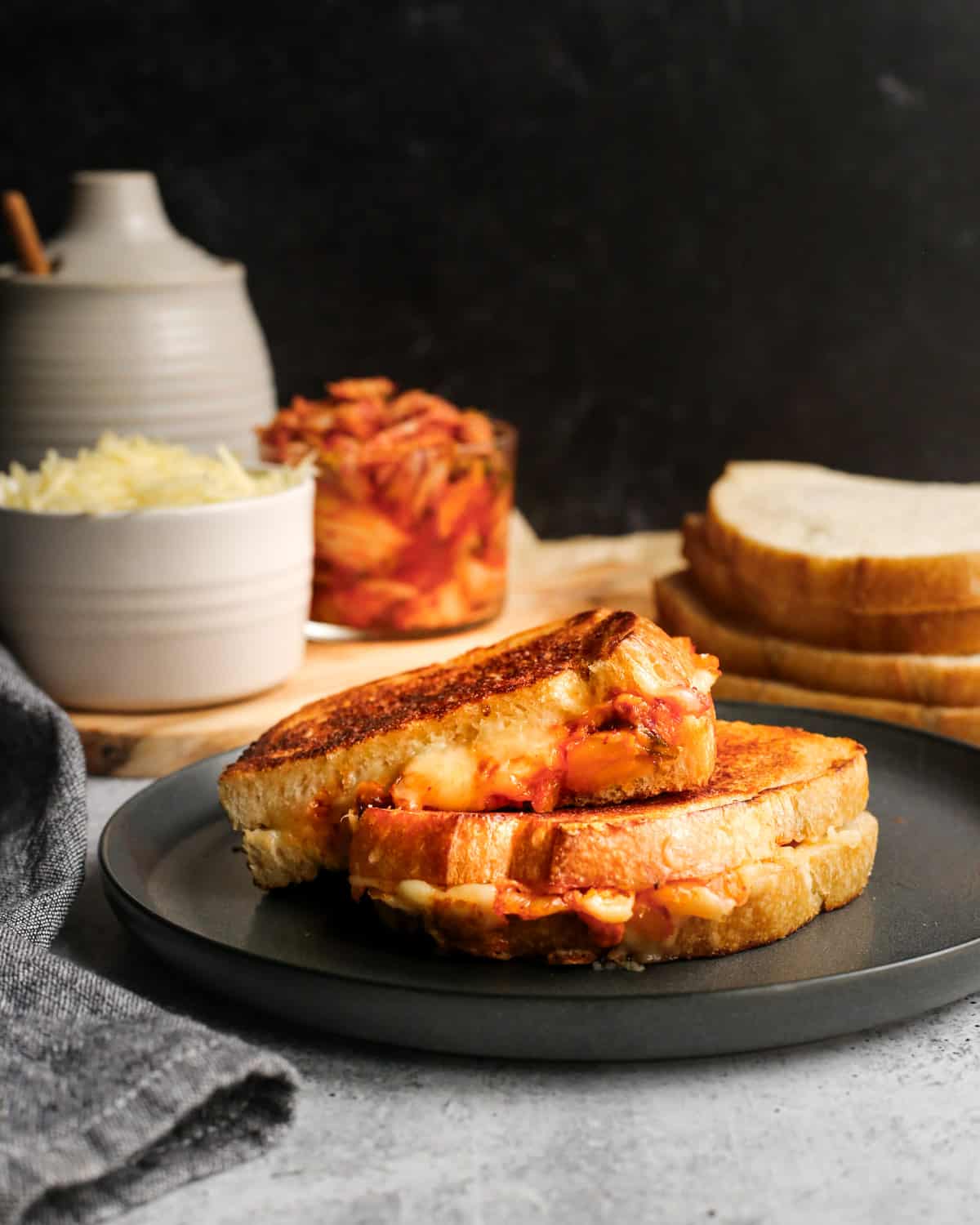This detailed indoor close-up photograph showcases a beautifully crafted grilled cheese sandwich placed on a flat, matte black plate in the foreground. The sandwich, made with thin artisanal bread, is cut in half with one half artfully angled atop the other, revealing perfectly melted cheese and a hint of crispy bacon spilling out. To the left of the plate, a partially visible folded gray napkin adds a touch of elegance to the composition.

In the background, plain slices of untoasted bread are stacked neatly on the right side. On the left, a serving tray holds a ceramic cup filled with grated cheese next to a cutting board. Behind this tray stands a clear cup containing either sliced carrots or bacon, adding a splash of color. Further behind, a taller jar with a spoon emerging from it sits beside a small ceramic bowl with a lid, all set against a dark backdrop that makes the foreground elements pop. Natural light gently illuminates the scene, making the image look like it could feature in a gourmet menu advertising a grilled cheese sandwich.